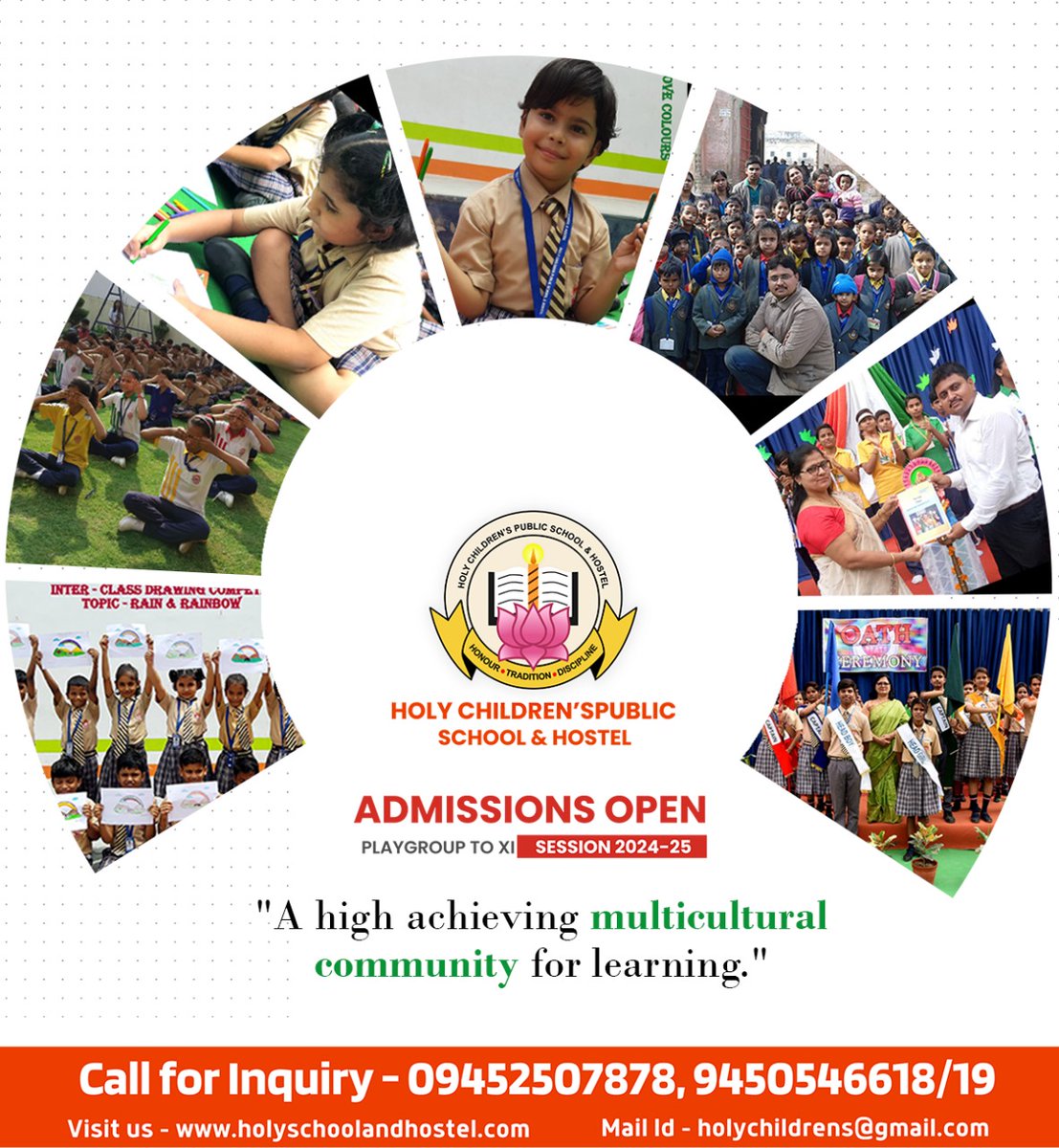This is an advertisement for Holy Children's Public School and Hostel, featuring a visually appealing, radial design. At the top, a pattern of small dots transitions into a two-thirds circular collage of seven photographs. These images showcase a diverse group of children and families engaging in various activities: children celebrating with medals, participating in outdoor exercises, working on art projects, receiving awards, and posing proudly with plaques and ribbons. The center of this circular arrangement prominently displays the school’s logo, which includes an open book with a candle and a small pink flower. The logo bears the institution's name, along with the slogan "Honor, Tradition, Discipline."

Below the logo, the flyer announces, "Admissions Open: Playgroup to XI Session 2024-2025," highlighting the school as a "high-achieving multicultural community for learning." For more information, the advertisement encourages viewers to call for inquiry, visit the school’s website at www.holyschoolandhostel.com, or email at holychildrens@gmail.com. This information is presented at the bottom of the flyer on an orange banner.